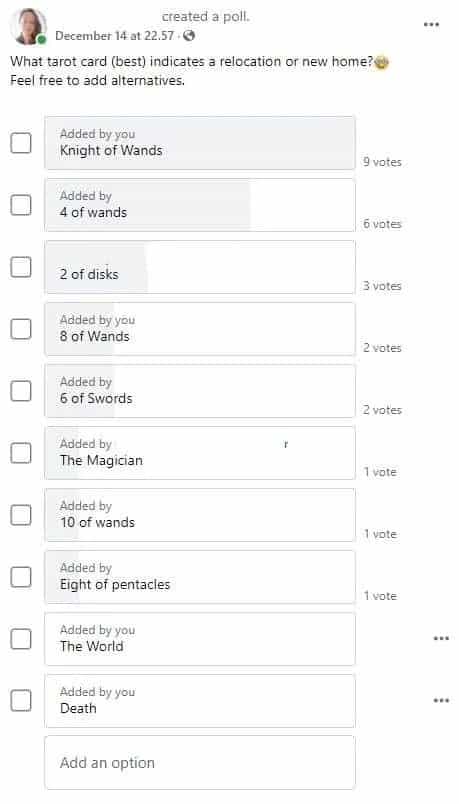In this image, we see a screenshot of a social media post featuring a poll conducted on December 14th at 10:57 PM. The poll seeks to determine which tarot card best symbolizes the idea of relocating to a new home. The question posed is: "Which tarot card best indicates a relocation or a new home? Feel free to add alternatives."

The options provided in the poll are as follows:
1. 9 of Wands
2. 4 of Wands
3. 2 of Discs
4. 8 of Wands
5. 6 of Swords
6. The Magician
7. 10 of Wands
8. 8 of Pentacles
9. The World
10. Death

Each option has garnered votes, with the 9 of Wands notably receiving 9 votes. The post reflects an engaging discussion among tarot enthusiasts, offering insight into the diverse interpretations of tarot cards related to the theme of moving to a new residence.